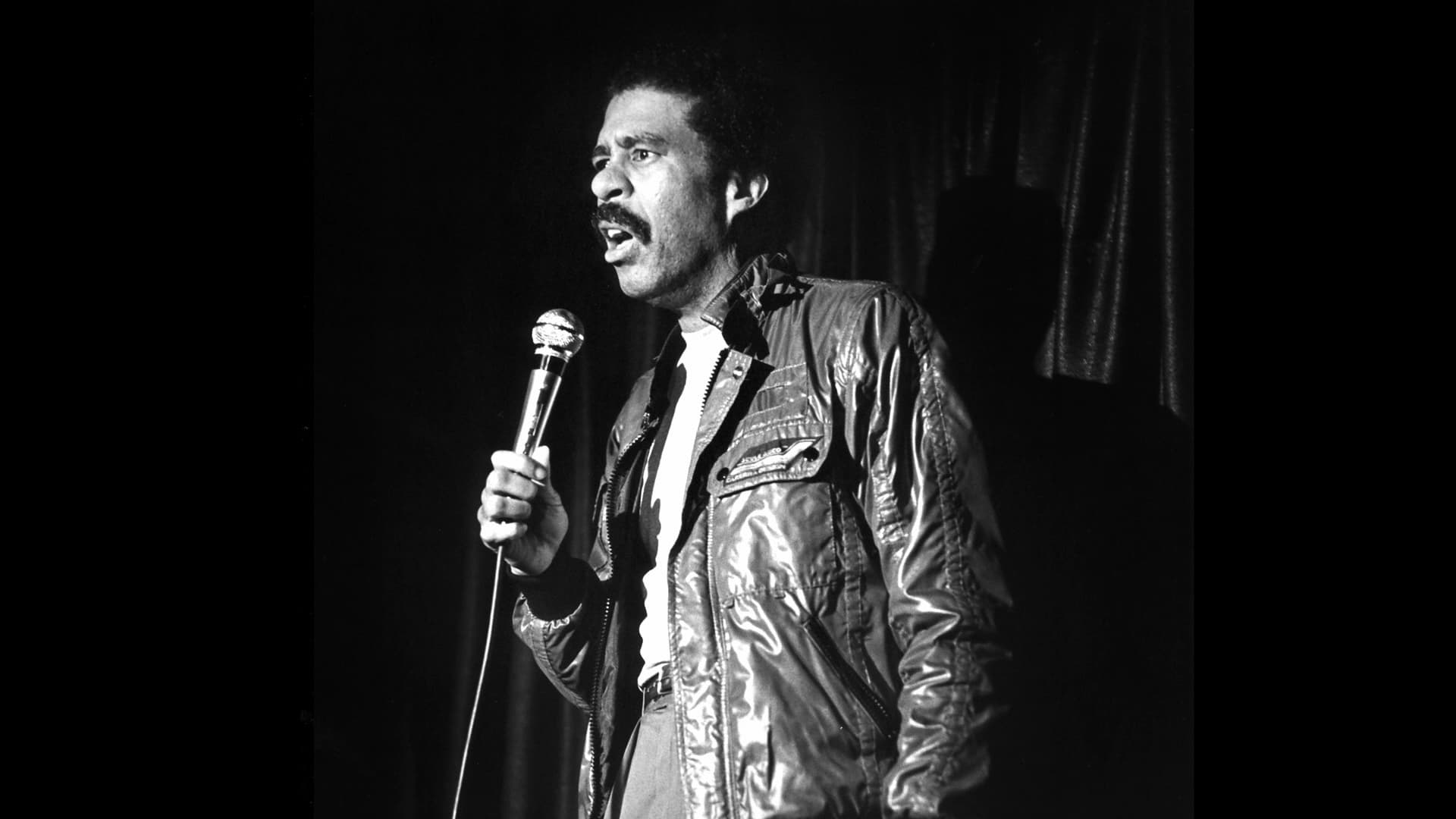This black-and-white photograph captures the iconic comedian Richard Pryor standing on a dimly lit stage, holding a large metal microphone in his right hand, which is raised to his mouth as he delivers a punchline. The solitary spotlight illuminates Pryor from the front, casting a crisp shadow of his head and shoulders against the ruffled backdrop of the stage curtain behind him. His facial expression is one of exaggerated exasperation, with his mouth open and laugh lines accentuating the corners of his eyes, reflecting his comedic performance. 

Pryor is dressed in a thick, open leather jacket that reveals a plain white t-shirt underneath. The waistband of his trousers and his belt are visible, but the image confines him to a waist-up view. His left hand rests casually by his side. Known for his expressive face and prominent mustache, the relatively small stature of Pryor is evident here. This compelling image epitomizes Pryor's commanding stage presence and his ability to engage audiences through physical expression in his stand-up routines.